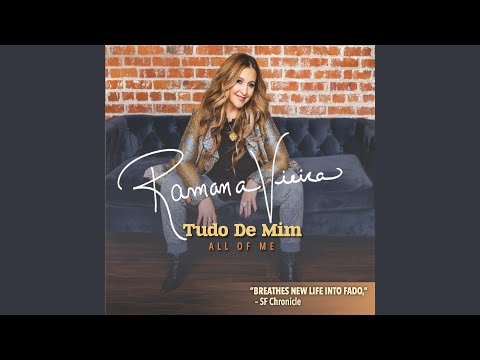The album cover features a young woman seated on a dark-colored, likely navy blue, velvet couch placed in front of a red brick wall. She has long, wavy brown hair cascading past her shoulders, and she is smiling directly at the camera. She wears a black top beneath a brown jacket, complemented by blue jeans and a necklace with a pendant. The text on the cover reads "Romana Vieira, Tudor de Mim," with the English translation "All of me" underneath. The bottom right corner of the cover features the phrase, "Breathes new life into Fado," attributed to the SF Chronicle. The image is bordered by black strips on the top and bottom and gray strips on the sides, and the entire setting is brightly lit and clearly visible.